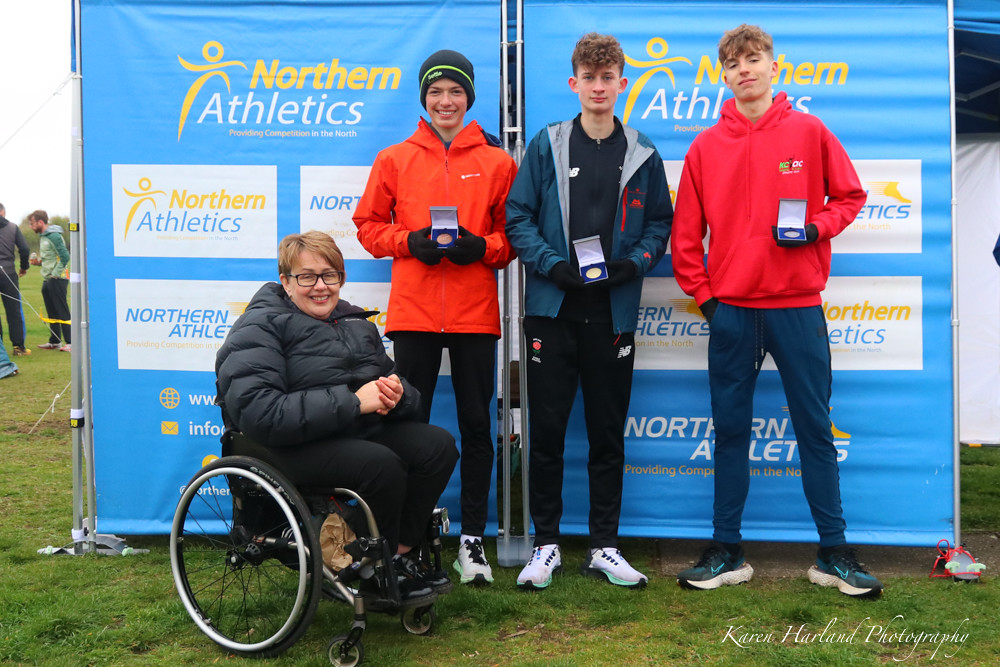The photograph depicts a group of four individuals posing in front of two identical light blue banners set in metal rectangular frames. The banners prominently feature multiple logos, with the top logo displaying the text "Northern" in yellow and "Athletics" in white. The tagline "providing competition in the north" is also visible. In the bottom right corner of the photograph, there is a cursive white watermark that reads "Karen Harland Photography."

From left to right, the people in the photograph are as follows: The first individual is a woman seated in a four-wheeled wheelchair, wearing glasses, black pants, and a black parka. Next to her stands a person in tight black pants, white tennis shoes, and an orange jacket zipped up, complemented by black gloves. This person is holding a small box, flipped open to reveal a gold medal. The remaining individuals, who appear to be teenagers, are also focused on showcasing these boxes that display gold medals.

All four individuals are facing forward, collectively highlighting their achievements, with the distinctive Northern Athletics banners serving as their backdrop.